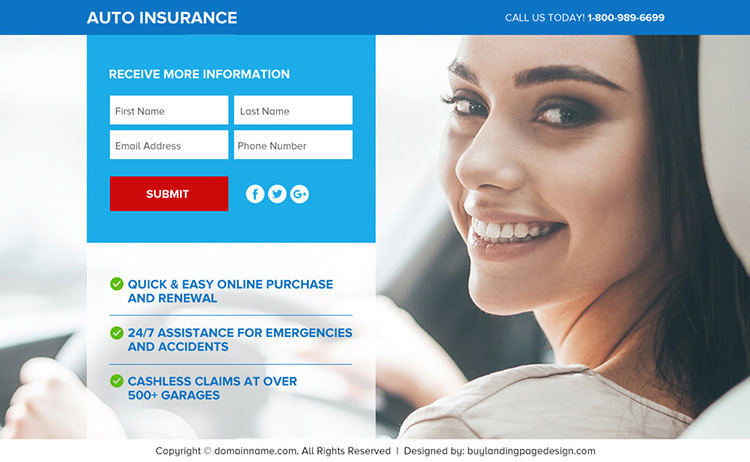The image features an informative advertisement for auto insurance services. At the top of the ad is a dark blue border, with the left side displaying "AUTO INSURANCE" in white capital letters, and the right side stating "Call us today: 1-800-989-6699." Below this is a light blue box with white capital letters that say, "RECEIVE MORE INFORMATION."

Inside the main content area, there is a form containing fields labeled "First Name," "Last Name," "Email Address," and "Phone Number." A red box with the word "SUBMIT" invites users to provide their details. Social media icons for Facebook, Twitter, and Google are situated underneath the submission button.

Further down, a white box features three green circles with check marks accompanied by text bullets: "Quick and easy online purchase and renewal," "24/7 assistance for emergencies and accidents," and "Cashless claim to over 500 garages."

On the right side of the advertisement, there is an image of a smiling woman, shown from her shoulders to her forehead, engaging directly with the camera. Finally, at the bottom of the ad, the text "© domainname.com All rights reserved" can be found.